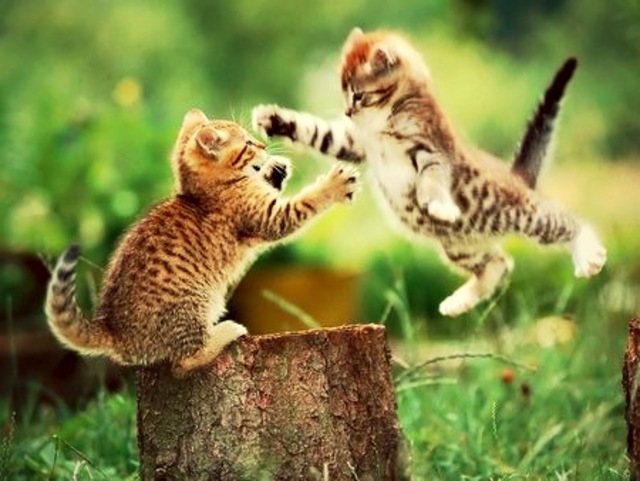In a sunlit field surrounded by blurry trees and tall grass, two playful kittens are captured mid-action. A small tree stump sits at the center of the image, with the left kitten's back legs firmly planted on it. This kitten, an orange and black striped feline with a black-tipped tail, has its front paws outstretched in the air, seemingly reaching for the other kitten. The right kitten, also striped but with a combination of orange and white, including a white tummy and paws, is airborne, flying towards the left kitten with its arms spread wide and its mostly black tail straight out. Their playful interaction is set against a backdrop that includes a few indistinct yellow flowers, pieces of wood on the lower left and right of the image, and a bright, clear day full of vivid colors – greens, yellows, browns, oranges, whites, and tans.